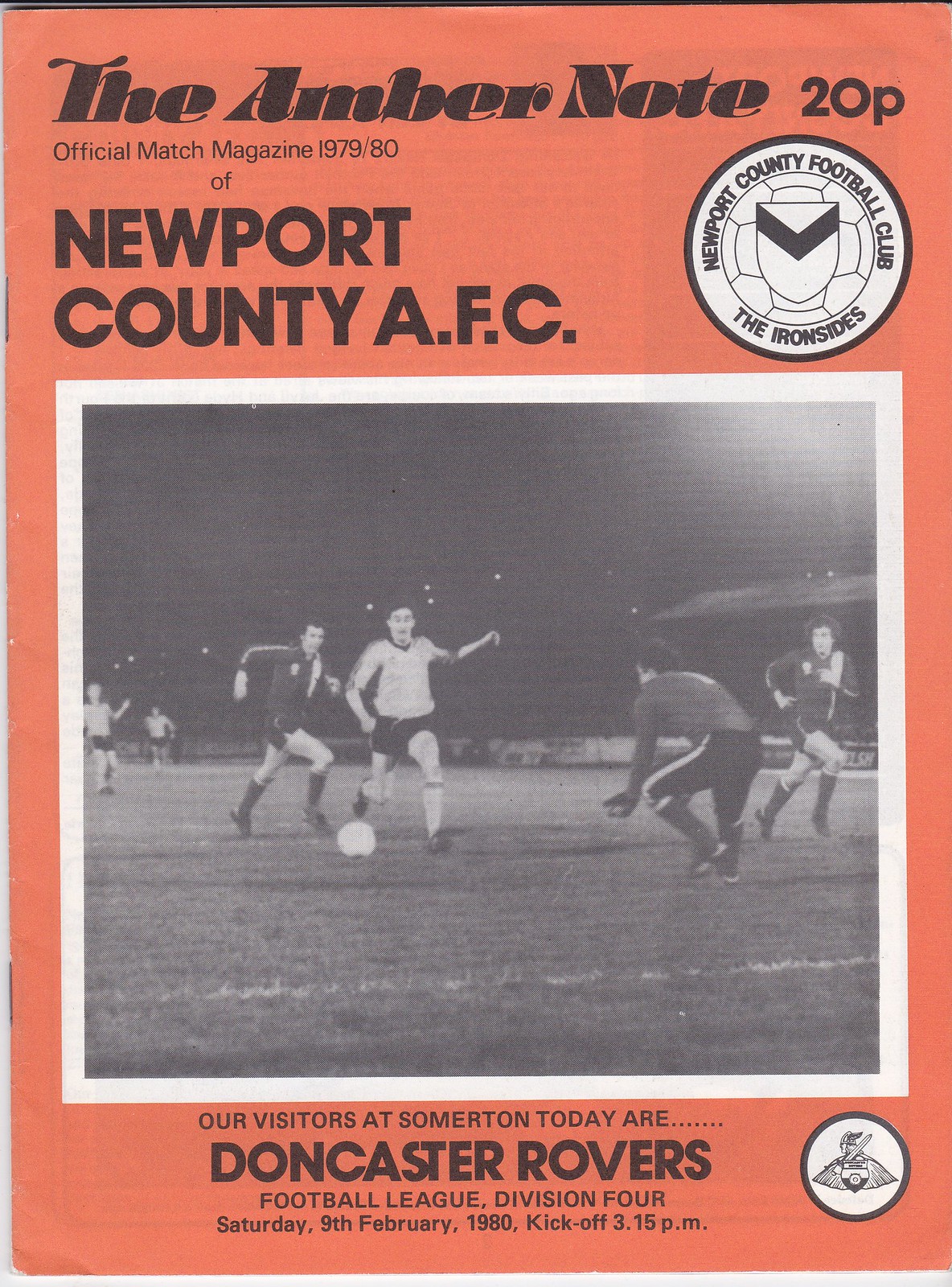The cover of the game day program for Newport County AFC's official match magazine from the 1979-1980 season features a vintage design with a rose-red background and black text. At the top, it reads "The Amber Note 20P," indicating the cost in pence. The Newport County AFC logo, depicted in black and white in a circular format, is positioned to the right of the heading. Central to the cover is a grainy, black and white action photograph capturing six players mid-game; players in white appear to be attacking, with one getting ready to shoot at the goal as the goalkeeper, arms down, prepares to defend, while a challenger approaches and another player is positioned behind the goalie. The game appears to be set outdoors at night. At the bottom, the text states "Our visitors at Somerton today are Doncaster Rovers, Football League, Division IV, Saturday, 9th February 1980, kickoff at 3.15 p.m." The cover incorporates additional colors of gray and white, enhancing its vintage appeal. The Doncaster Rovers mascot is also depicted within a circle to the right of the event details.